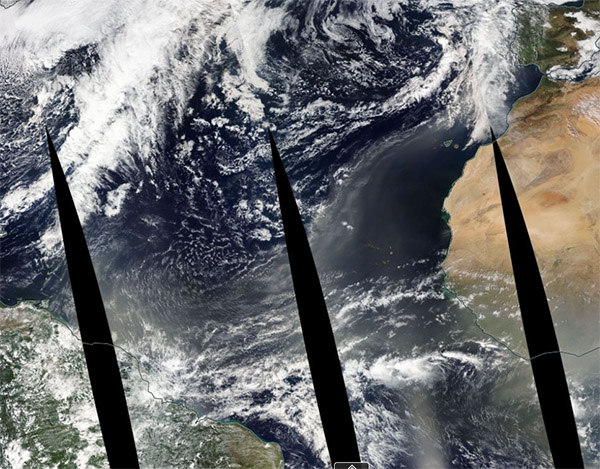This horizontal, rectangular satellite image captures a dynamic scene from space, revealing swirling black storm clouds with prominent white edges, suggestive of a powerful cyclone or hurricane. The image distinctly shows the Earth's surface below, where brown farm fields, blue oceans, and green vegetative patches are visible. A portion of a continent, possibly Africa with its sandy stretches, is also discernible. In the forefront, three vertical, black, conical-shaped structures or shadows, which might be parts of the satellite or perhaps a wrought iron fence with pointed tops, are prominently positioned, providing a stark contrast against the tumultuous weather patterns and geographical features below. The overall view emphasizes the vastness and intricate details of the Earth's surface and atmosphere from a top-down perspective.